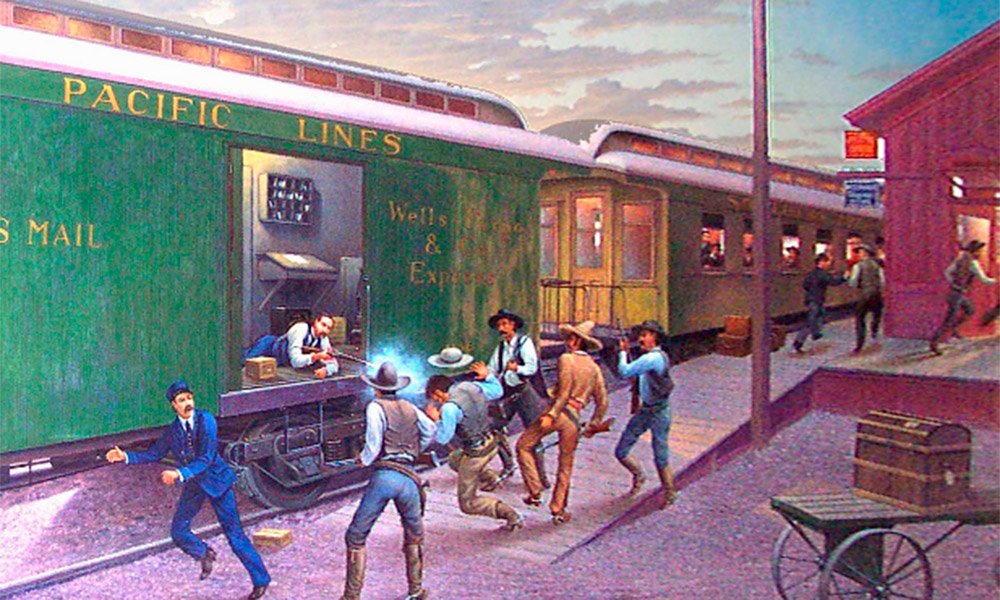The image is a detailed colored print or painting depicting an intense scene at a Western railroad station during what appears to be a train robbery attempt. In the foreground, a green Pacific Lines and Wells Fargo express car, identifiable by its label, dominates the approach from the left side of the image, extending towards the middle. The train is stationary by a wooden, red train depot located in the far right corner. The sky fades from a pinkish tone to a blue with clouds, indicating it is evening. A wooden platform is visible, bustling with activity.

A dramatic standoff is unfolding: a train employee, partly out a window of the express car, is wielding a shotgun and firing at a group of approximately six cowboys gathered near the open door of the car. The cowboys, all with their backs to the viewer, include men in classic cowboy hats, an individual in a Mexican cowboy outfit, and two men in black hats. One wounded cowboy appears to be falling. Amidst this chaotic scene, a train conductor is seen fleeing to the left, adding to the sense of urgency.

People on the platform are also depicted in a state of panic, running away from the scene, and in the lower right corner, there's a baggage cart. The background also shows a purplish-red sky, enhancing the dramatic atmosphere of the attempted heist gone awry. This richly detailed image captures the chaos and tension of a thwarted train robbery in the Old West, complete with vivid characters and atmospheric details.